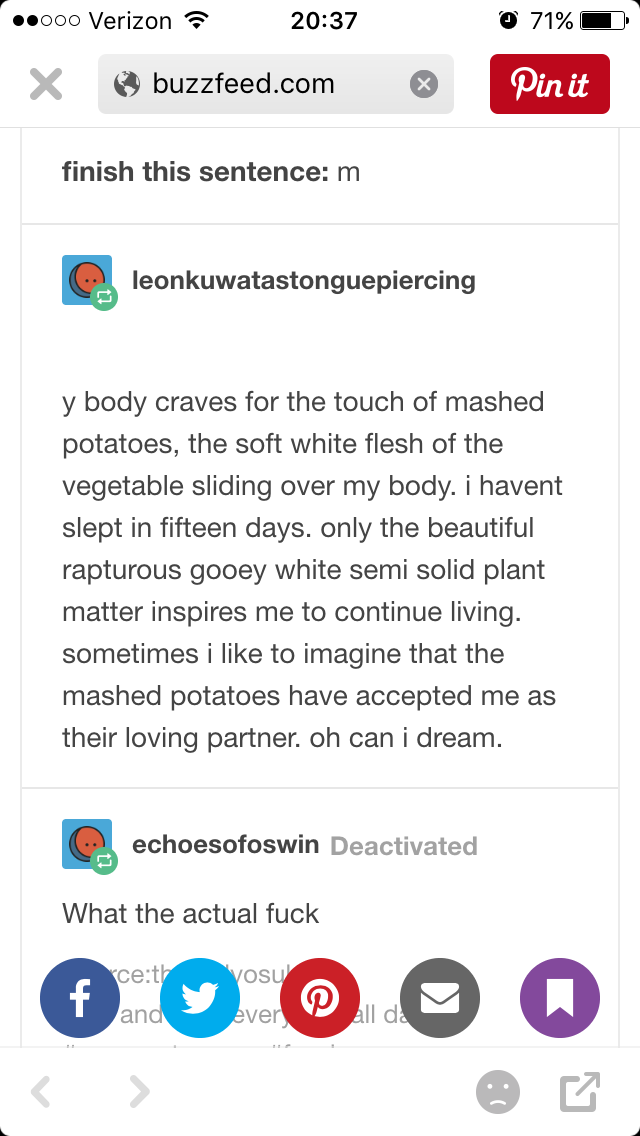This is a detailed screenshot taken from a smartphone, evident from the familiar icons along the top: a battery indicator showing 71%, a small alarm clock symbol with white hands, the time displayed as 20:37, a Wi-Fi symbol resembling a series of concave lines growing larger upward, and the carrier name "Verizon" next to it. Below these, a gray rectangle with a globe icon contains the URL "buzzfeed.com", and to its right, a red "Pin It" button for Pinterest. Along the bottom, there are equally sized and spaced icons for social sharing: Facebook (a white "f" on blue), Twitter (a white bird on blue), Pinterest (a red logo), Email (a white envelope on gray), and a bookmarking tool (a white bookmark on purple). The main content displays an article titled "Finish this sentence: M" featuring user comments. Prominently, it includes a bizarre and humorous post by Leon Kuwada Stong-Piercing about an obsessive craving for mashed potatoes, describing an odd fantasy about mashed potatoes that serves as a comedic element in the screenshot from BuzzFeed.com.